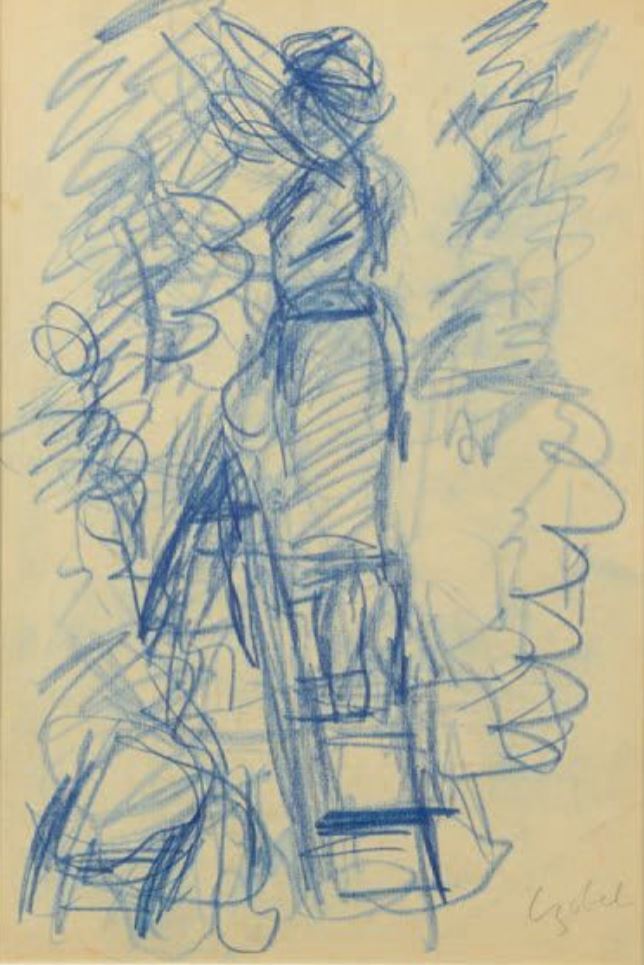This is an abstract sketch drawing, seemingly created with a blue-colored pencil or soft medium like charcoal or crayon, on manila or tan paper. The image depicts a woman with her hair up in a bun, standing on the second rung of a step ladder, which does not show its top. The woman is dressed in an apron that features pockets or items, possibly a wash rag, hanging from it. She appears to be barefoot with her legs exposed. Although the lines are squiggly and give an amateurish feel, the figure's shape, including curves and a slightly defined head, suggest it's a woman. The background is filled with energetic, almost violent scribbles, including M-shaped lines and other random patterns, which convey a sense of motion, as if the woman might be painting a wall.